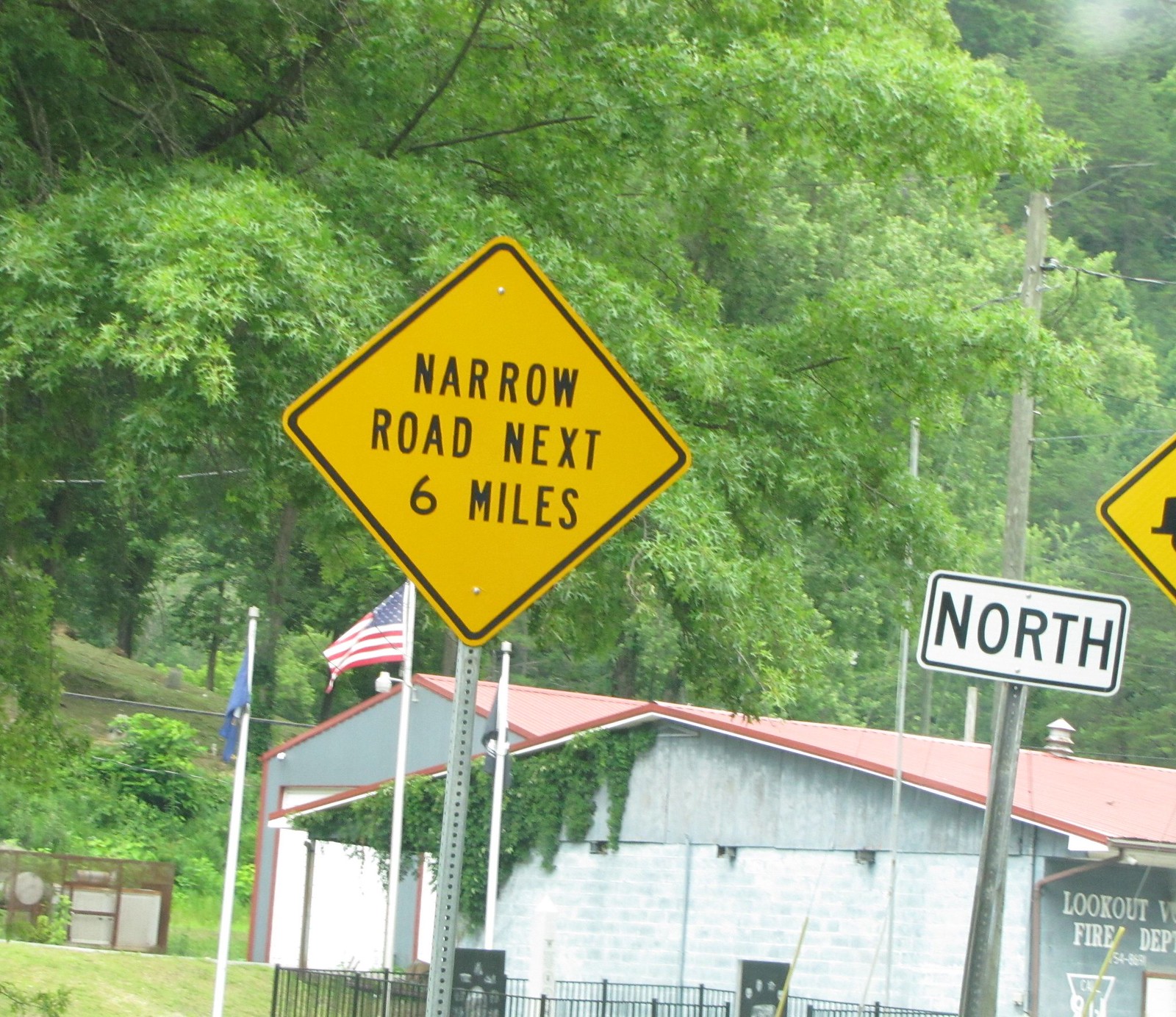The image is a large, vertical outdoor photograph capturing a scenic, slightly inclined landscape. In the background, a series of trees ascend, suggesting a hilly terrain. Below, a gray building with a red roof stands prominently. Surrounding the building are various power lines and flags, including the American flag and a blue flag, both fluttering energetically in the wind. The building, identified as a part of the local fire department, is enclosed by a black fence. Several street signs are visible: one yellow sign with black lettering warns "Narrow Road, Next 6 Miles," and another sign in white with black letters indicates "North."